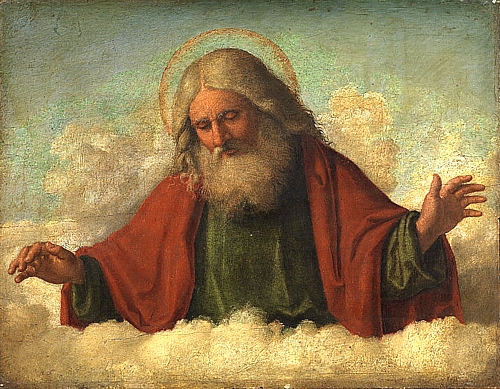The image depicts a detailed, vintage artwork with a religious theme, reminiscent of illustrations from an older Bible. Central to the piece is a white-haired, white-bearded man, exuding an air of divinity, potentially representing God or Jesus. His long, flowing hair is parted in the middle, accompanied by a bushy beard and an impressive handlebar mustache. The man is dressed in a red robe or mantle draped over an olive green tunic, extending his hands outward. His face is tipped downwards and toward the left corner of the image, enhancing a contemplative expression. Enhancing his divine aura is a faint, golden halo that crowns his head. He appears to be emerging above a layer of fluffy, muted clouds in tans and beiges, set against a backdrop of a sea-green sky, creating a celestial atmosphere. His demeanor and the overall composition suggest he is gazing down, perhaps observing or blessing the world below.